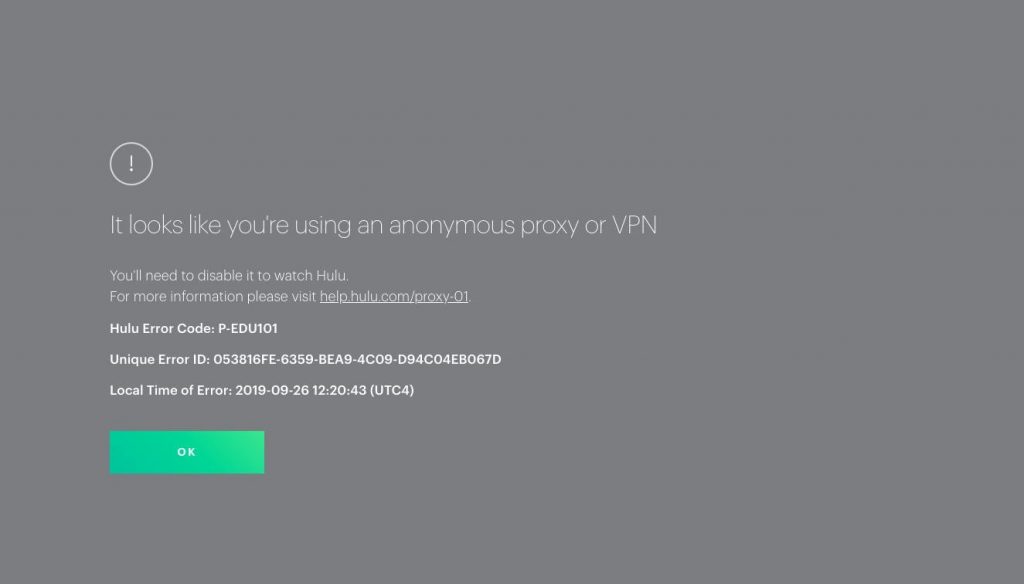The image depicts a grey notification box displayed by Hulu, indicating that the user is attempting to access the service via an anonymous proxy or VPN. The alert features a prominent exclamation mark within a white circle, accompanied by the message informing the user that they must disable their proxy or VPN to continue using Hulu. The text directs users seeking further information to visit help.hulu.com/proxy-o-1. The error is identified as Hulu Error Code P-EDU101, with a Unique Error ID of 053816FE-6359-BEA9-4C09-D94C04EB067D. The specific time of the error occurrence is stated as 2019-09-26 at 12:20:43 UTC-4. Below this detailed information, there is a green "OK" button for users to acknowledge the message. This notification highlights the inconvenience faced by subscribers who are unable to access Hulu while using a VPN despite having a valid subscription.